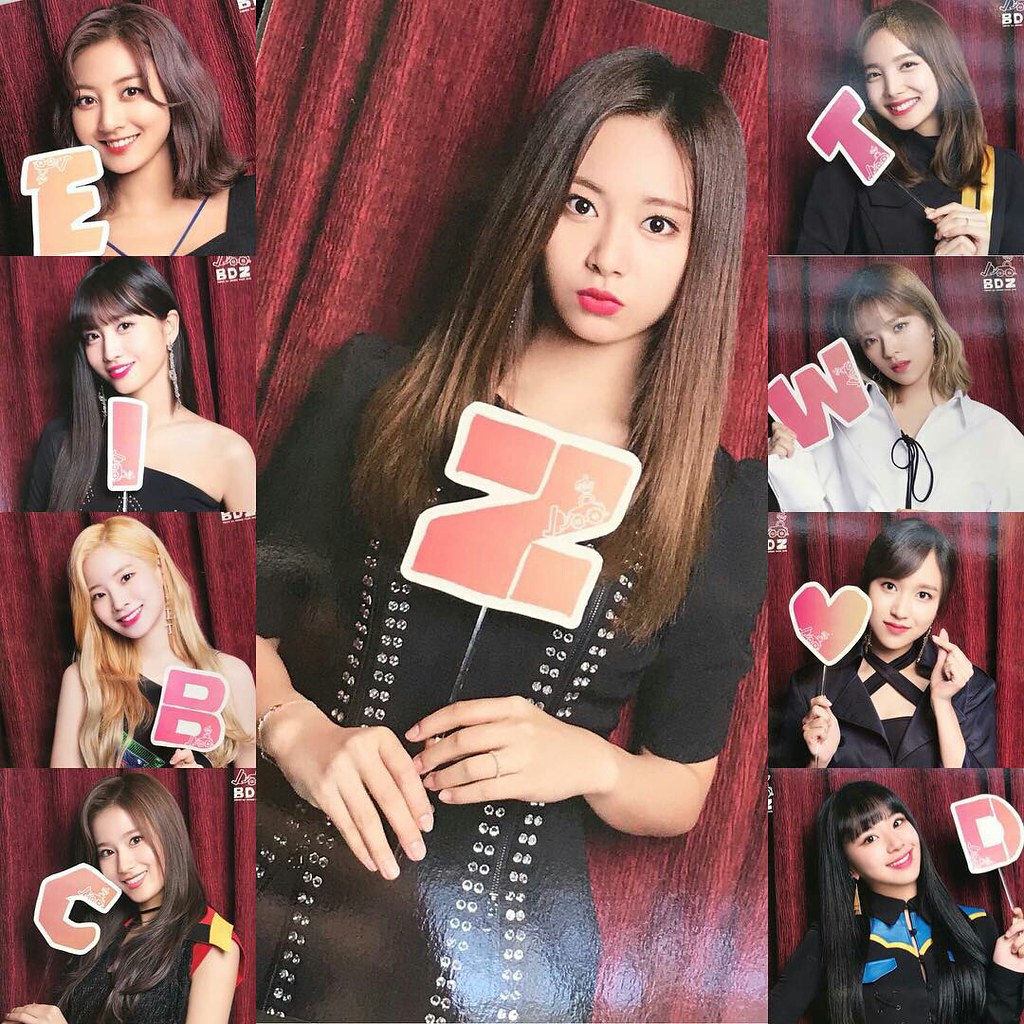In a vibrant photo booth collage, centered prominently is an 18-year-old Asian girl with straight brown hair and pink lipstick, wearing a black dress adorned with silver rivets. She pouts playfully at the camera while holding a red "Z." Surrounding her, against a rich maroon curtain backdrop, are eight smaller photos of other young Asian girls, each holding different letters or a heart. The sequence of letters along the left side is "E," "I," "B," and "C," while on the right it is "T," "W," a heart, and "D." Most of the girls are dressed in black, with a mix of red, yellow, and white accents. The variations in hair color and outfits across the photos add a dynamic and cohesive feel to the collage, enhancing the playful and coordinated theme of the shoot.